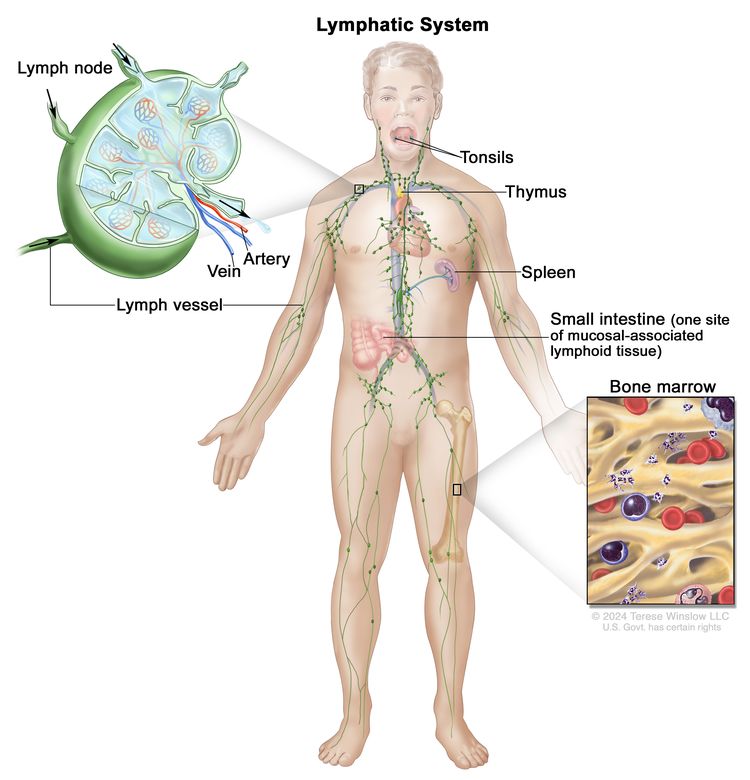This digital drawing illustrates the lymphatic system of a human male, depicted with arms outstretched. The title "Lymphatic System" is prominently displayed at the top in black text. Across the body, green lines and dots indicate the lymphatic vessels and structures. Key features are labeled: tonsils, thymus, spleen, and small intestines, identified as part of the mucosal-associated lymphoid tissue. On the left, a detailed inset shows a cross-section of a lymph node, annotated to indicate where veins and arteries enter. Another inset on the bottom right presents a close-up of bone marrow, showing red blood cells and another type of cell in purple. The image includes color-coded details, featuring hues of yellowish beige, red, pink, purple, green, light blue, and black. Finally, beneath the bone marrow illustration, a copyright notice states: "2024, Teresa Wilson, LLC, U.S. government has certain rights."